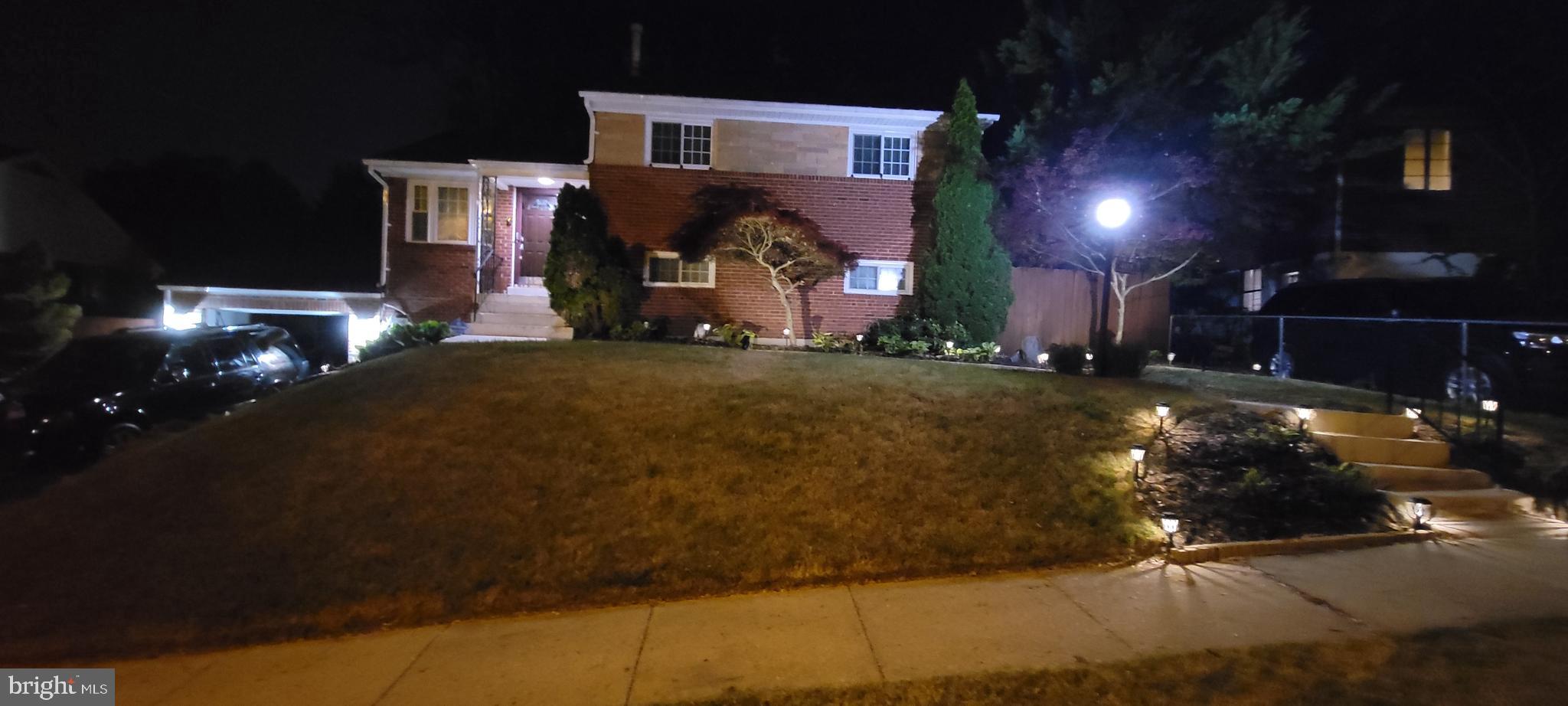The nighttime photograph captures a two-story house perched on a sloping hill. The house features a striking combination of red brick on the bottom story and beige brick with white accents on the top story. Illuminated by an array of lights, including small stake lights along the winding walkway and additional lights on the ceiling and the garage, the house glows warmly in the night. A large lamppost stands to the right, casting light over the scene, while a tall tree looms behind it. The driveway and garage are located on the left side, with the garage flanked by lamps. Steps meander up the hill, first approaching and then leading up to the front door. A chain link fence lines the right edge of the property. The grass appears brownish-green, contrasting with the level paved sidewalk at the bottom of the slope.